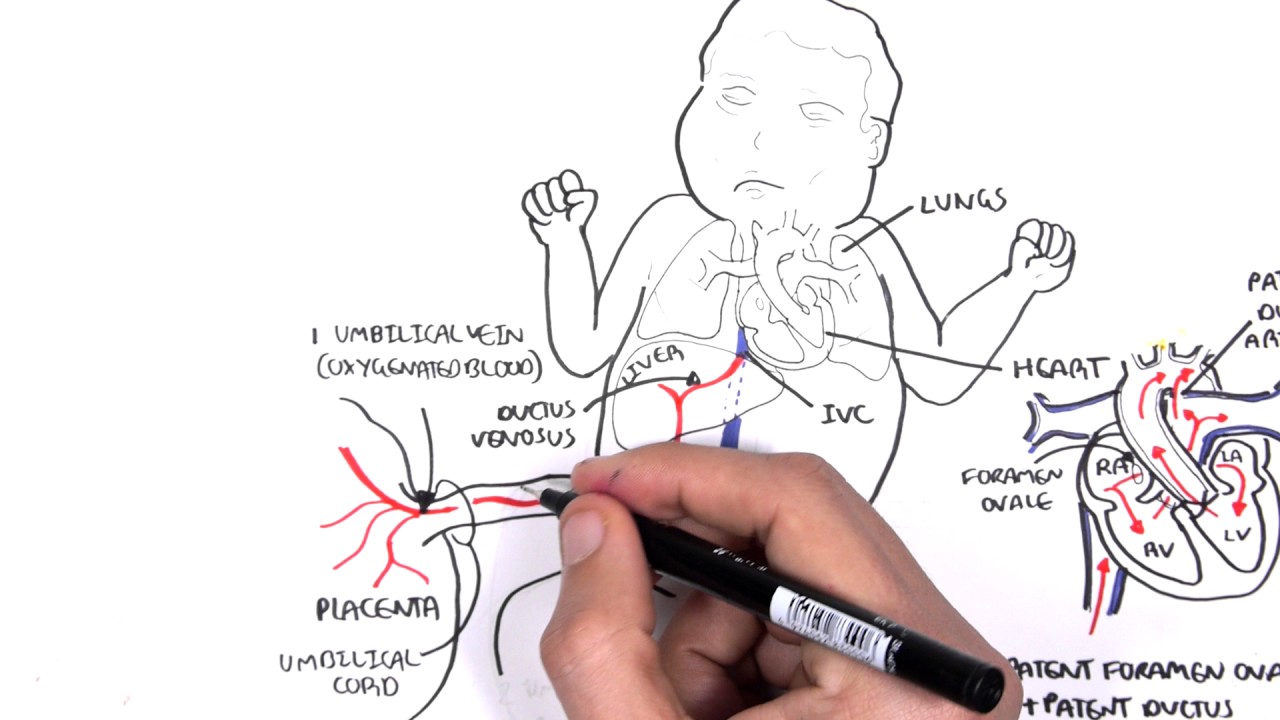The image depicts a detailed illustration, either hand-drawn or digitally rendered to mimic the appearance of a hand drawing. At the bottom of the image, a male hand holds a black pen, likely a marker, poised against the paper, actively drawing the illustration. The central subject of the drawing is a baby, with its arms raised, showcasing various internal organs labeled with precise annotations. Visible organs include the lungs, heart, liver, and IVC (Inferior Vena Cava). The labels are connected to the corresponding parts via lines.

The right side of the image features a close-up of the heart, marked with terms such as "foramen ovale," "RV," "LV," "LA," and "RA," along with small red arrows indicating the blood flow. Below these details, the phrase "patent formation" appears, though it is partially cut off.

On the left side, additional annotations and diagrams elaborate on elements like the umbilical vein (depicted with red color to indicate oxygenated blood) and the ductus venosus. Further to the left, another drawing illustrates the placenta and umbilical cord. The entire image is rendered predominantly in black and white, with selective use of flesh tones, blue, and red to highlight specific anatomical details.